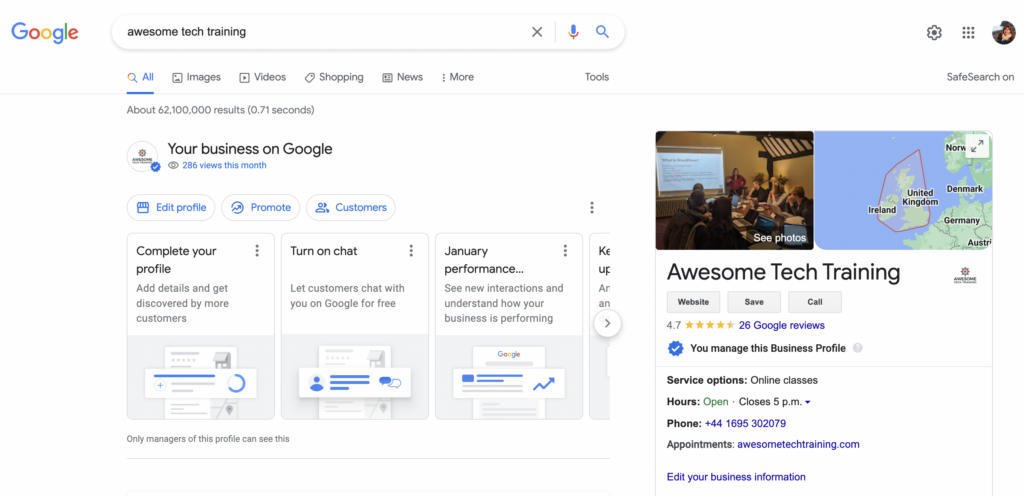The image depicts a Google search results page with the classic rainbow Google logo positioned on the top left. To the right of the logo, the user has conducted a search for "Awesome Tech Training." Adjacent to the search query, there's an 'X' icon for clearing the text, a microphone icon for voice input, a magnifying glass for search functionality, and a cogwheel icon for settings. Additionally, there are six or nine-dot icons that provide access to other Google apps, and a user profile circle that indicates "SafeSearch" is turned on.

Directly under the search bar, the "All" tab is highlighted, indicating the current search mode, with other options including Images, Videos, Shopping, News, More, and Tools. The search has yielded approximately 62 million results in less than a second. Underneath this, there's a section titled "Your Business on Google" displayed in bold black with a checkmark and a logo to the left, indicating that the business profile has 286 views this month. The headline is in blue, followed by options such as Edit Profile, Promote, and Customers.

Below this are four boxes, though only three are fully visible. The first box prompts users to complete their profile with "Add details and get discovered by more customers." A "Turn on chat" option is also present, allowing customers to communicate via Google for free. General performance metrics such as new interactions and business understanding are included.

To the right section, there is a detailed view of the "Awesome Tech Training" business profile, featuring options to visit the website, save the profile, or make a call. A Google review is also present, along with service options, hours of operation, phone number, and website. There's an option to edit these details. At the top, a featured image shows people engaged in a business meeting, while a map on the right indicates the business location somewhere between Ireland and the United Kingdom in Europe.